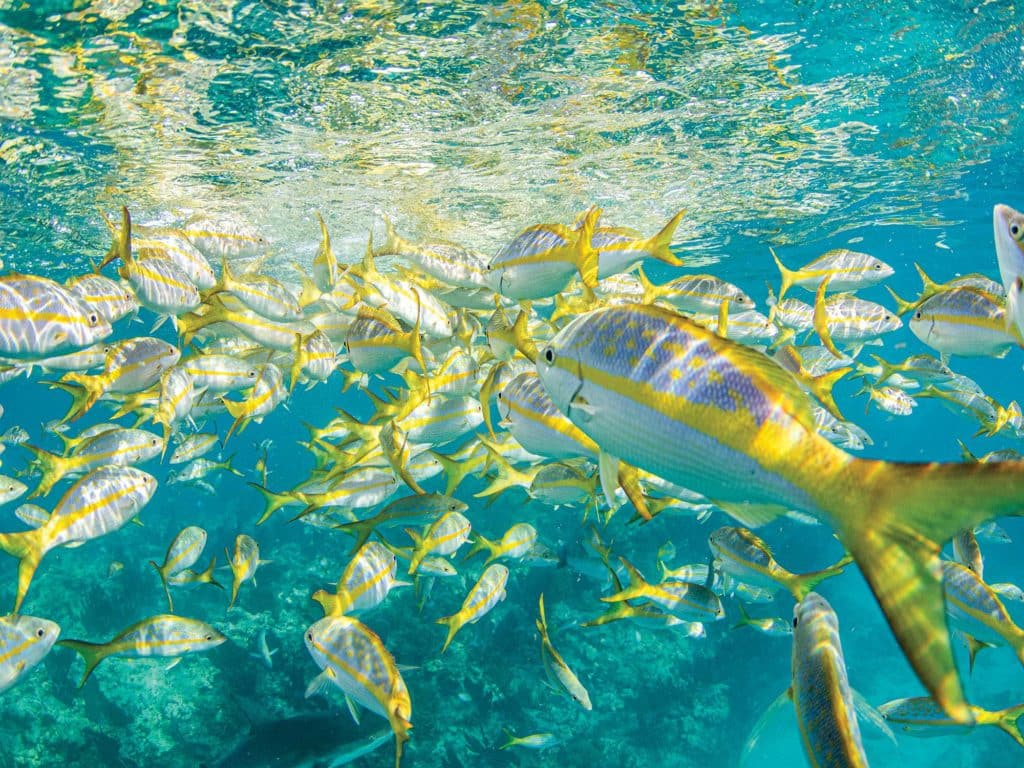The underwater photograph captures a vibrant and bustling underwater scene, presumably in the Caribbean or the Bahamas, featuring a large school of snappers. The fish, numbering around 50 to several hundred, all display a striking pattern with white bodies and yellow stripes running along their sides, complemented by yellow tails and occasional yellow spots on their upper halves. The water is a stunning Caribbean blue, and reflections of the fish are visible on the surface above, adding to the enchanting atmosphere. The fish appear to swim in unison, heading away from the camera. On the right side of the image, a prominent fish is close to the lens, showcasing the vivid details of its yellow stripe and tail. Beneath the school of fish, the ocean floor is visible, marked by grayish coral formations and rocks. The sunlight streaming from above interacts with the water, creating a dynamic play of light and color in the scene.